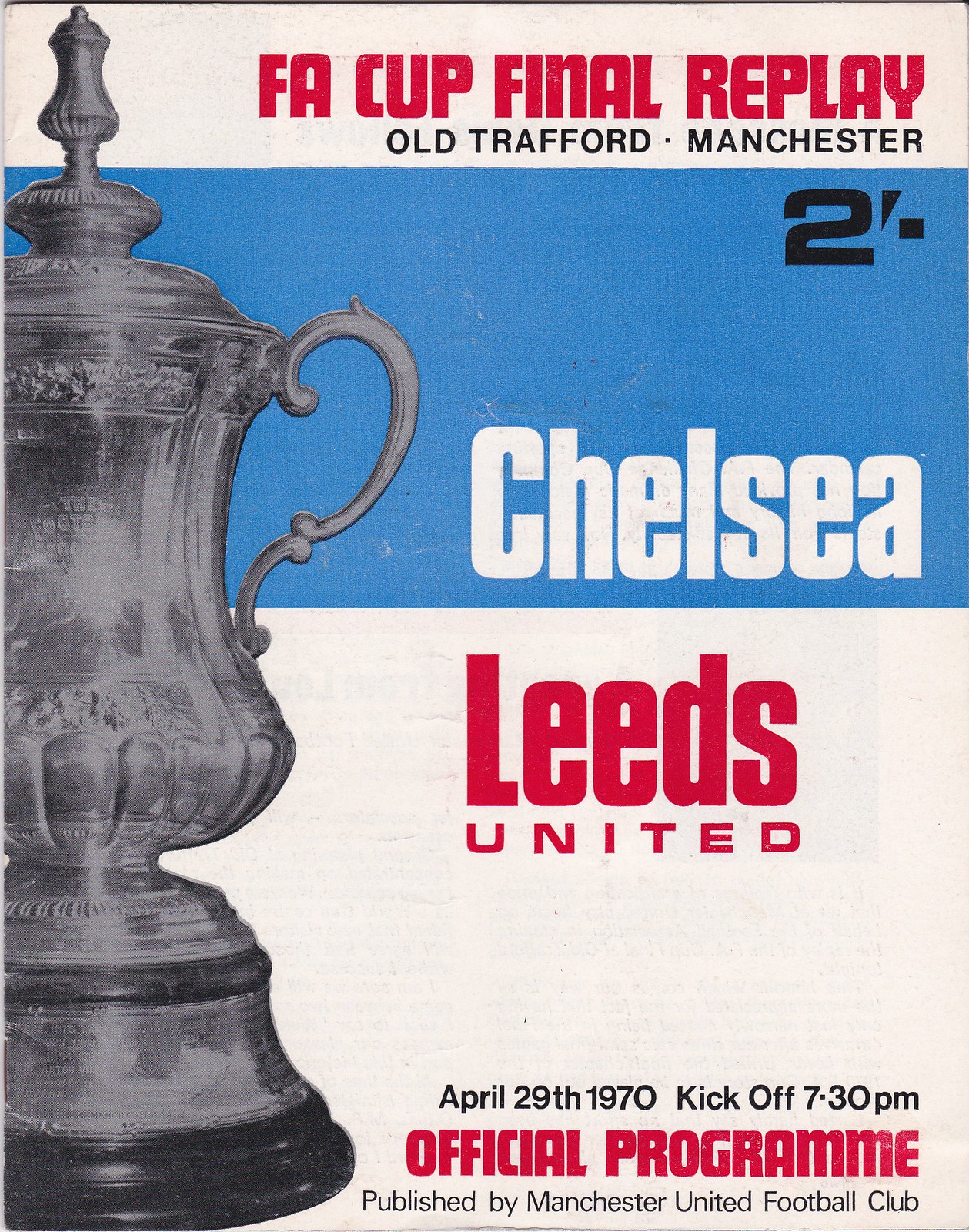This is the cover of an official program for the FA Cup Final Replay held on April 29, 1970, at Old Trafford, Manchester. The top of the poster features a white rectangular area with bold red text announcing "FA Cup Final Replay" and "Old Trafford, Manchester." Below this, a larger blue rectangular section prominently displays "Chelsea" in white letters, with the number two in black positioned at the top right corner. The bottom half of the cover is predominantly white, with red text stating "Leeds United Official Program" and black text providing the date and kickoff time: "April 29, 1970, kickoff 7.30 p.m." At the very bottom, in black letters, it indicates that the program is "published by Manchester United Football Club." To the left side of the cover, a gray and black image of the FA Cup trophy is visible, covering about three-quarters of the height, partially cut off on the left edge. The trophy appears intricate, showing a black base, handles, and a pointed top, adding a classic touch to the program's design.